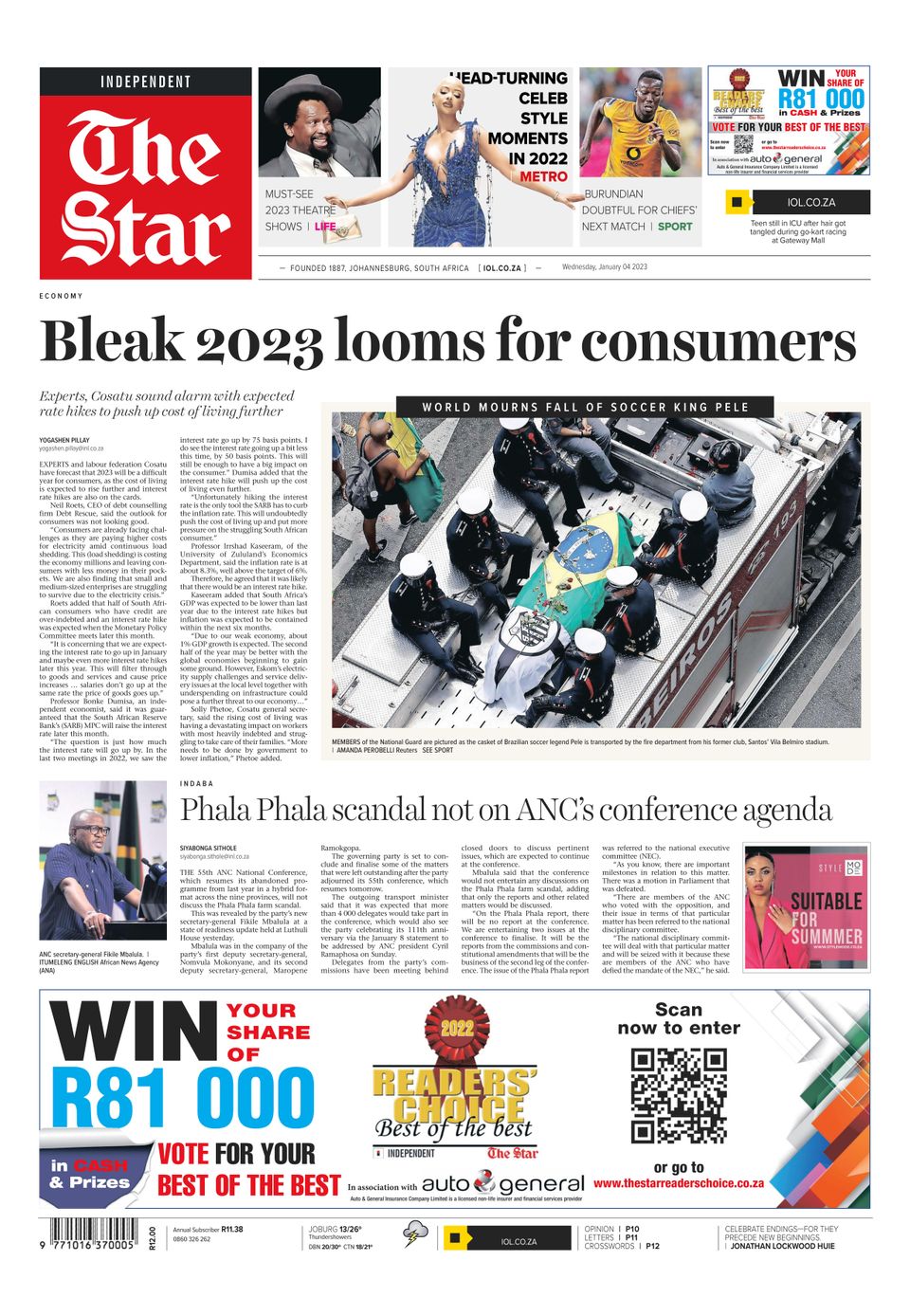**Detailed Caption:**

The front page of the featured newspaper is adorned with vibrant and attention-grabbing elements. In the upper left corner, a prominent black box with the word "Independent" boldly printed in white commands attention. Beneath it lies a striking red block with "The Star" inscribed in crisp white font. Running across the top of the newspaper, several photographs are displayed in a neat row. One image features a black man dressed impeccably in a gray suit and matching hat, with his hand raised. Adjacent to this is a segment titled "Head-Turning Celeb Style Moments in 2022," showcasing a blonde woman elegantly dressed in an elaborate blue gown. Further along, there is a picture of another black man participating in a marathon. The banner also mentions a chance to win R-8100, with a small black strip beneath declaring content "In Color."

The prominent headline "Bleak 2023 Looms for Consumers" takes center stage below these images. Accompanying the headline is a secondary lead, "World Mourns Fall of Soccer King," illustrated by a poignant photograph depicting uniformed men surrounding a casket draped in white, blue, and green, which is being carried atop a truck.

Another notable article headline, "Fela Fela Scandal Not on ANC's Conference Agenda," features an image of a gentleman involved in the relevant news. Adjacent to this, a bright pink block advertises "Suitable for the Summer" alongside a woman's picture. This section also entices readers with a chance to "Win Your Share of R-8100.”

Further down, the enticing call to action "Vote for Your Best of the Best" is prominently displayed, with "Vote" and "Best of the Best" highlighted in vibrant red. A small purple flag and a red ribbon labeled "Readers Choice" add to the decorative elements. Completing the front page, multiple colorful ribbons in green, orange, blue, pink, and white, along with a scannable code, hang down decoratively.